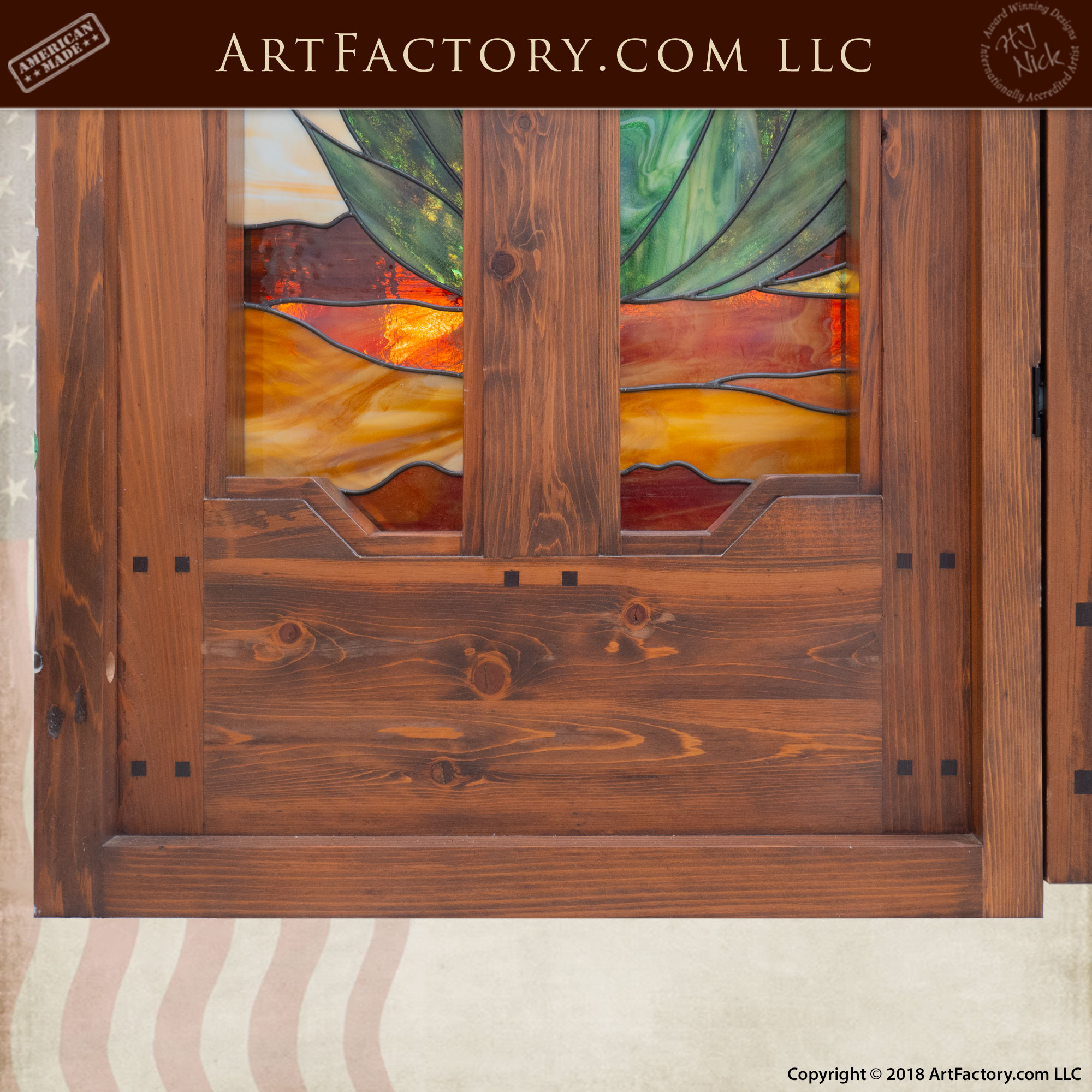The image depicts an advertisement for the website ArtFactory.com LLC, prominently featuring a doorway crafted from dark, stained wood. Central to the composition is a door-like structure, flanked on either side by vibrant stained glass panels. These panels showcase intricate designs of green leaves amidst swatches of orange, yellow, red, and hints of blue, creating a rich tapestry of colors including oranges, reds, greens, browns, beige, light pink, black, whites, and grays. A wooden partition runs vertically through the middle, separating the stained glass sections. Notable features include black squares and a hinge visible toward the bottom right of the door frame. The advertisement contains text in a brown border at the top stating "American Made" on the left and "ArtFactory.com LLC" in the center. The bottom right corner features a copyright notice: "Copyright 2018, ArtFactory.com LLC". This visual is presumably set within the context of the ArtFactory.com website.